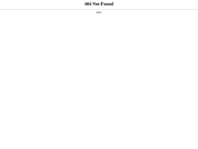The image depicts a minimalistic, white background with a central focus on three main elements: a line of text, a thin gray horizontal line, and a small gray splotch. At the top of the white screen, there is black text consisting of three words, with the last word appearing to be "found." However, the black text is very small and blurry, making it illegible. Directly beneath this text is a thin gray line, which spans approximately six times the width of the black text, also centered on the screen. Below this line, a small gray splotch can be observed, also centrally aligned with the other elements. These features are the only items on the otherwise plain white background, creating a simple and clean visual layout.